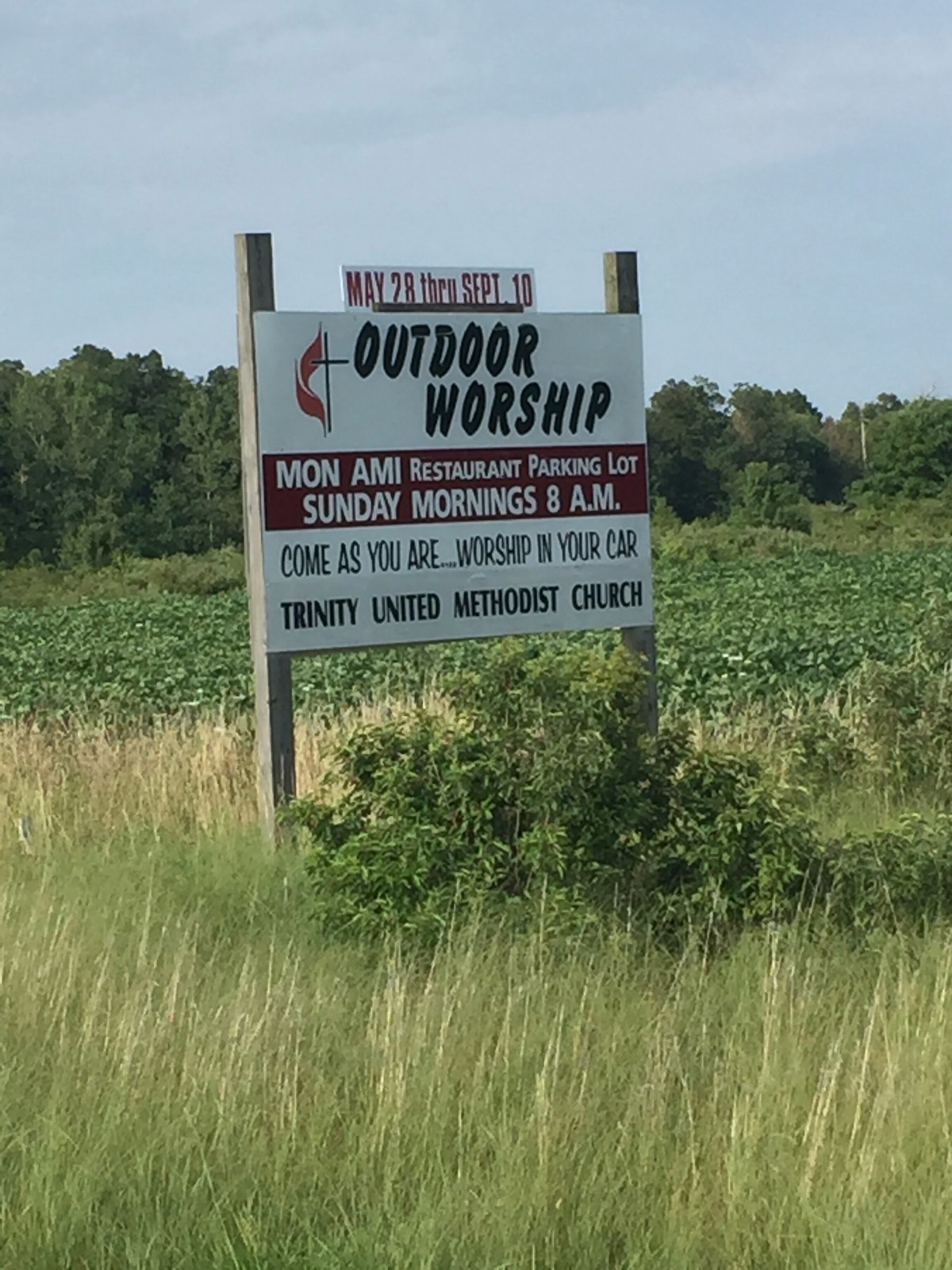Nestled in a picturesque field with tall yellow and green grass, stands a small but noticeable sign anchored between two wooden poles. This white sign with black and red lettering announces an opportunity for "Outdoor Worship" from "May 28th through September 10th" at the "Monomai Restaurant parking lot" on "Sunday mornings at 8 AM." The message invites passing drivers to "Come as you are" and "Worship in your car," courtesy of the "Trinity United Methodist Church." Behind the sign, which is partially obscured by a small bush and planted among rows of crops, the scene extends to a distant line of lush green trees beneath a typically overcast sky. The simple, modest sign effectively communicates its welcoming message to all who pass by.